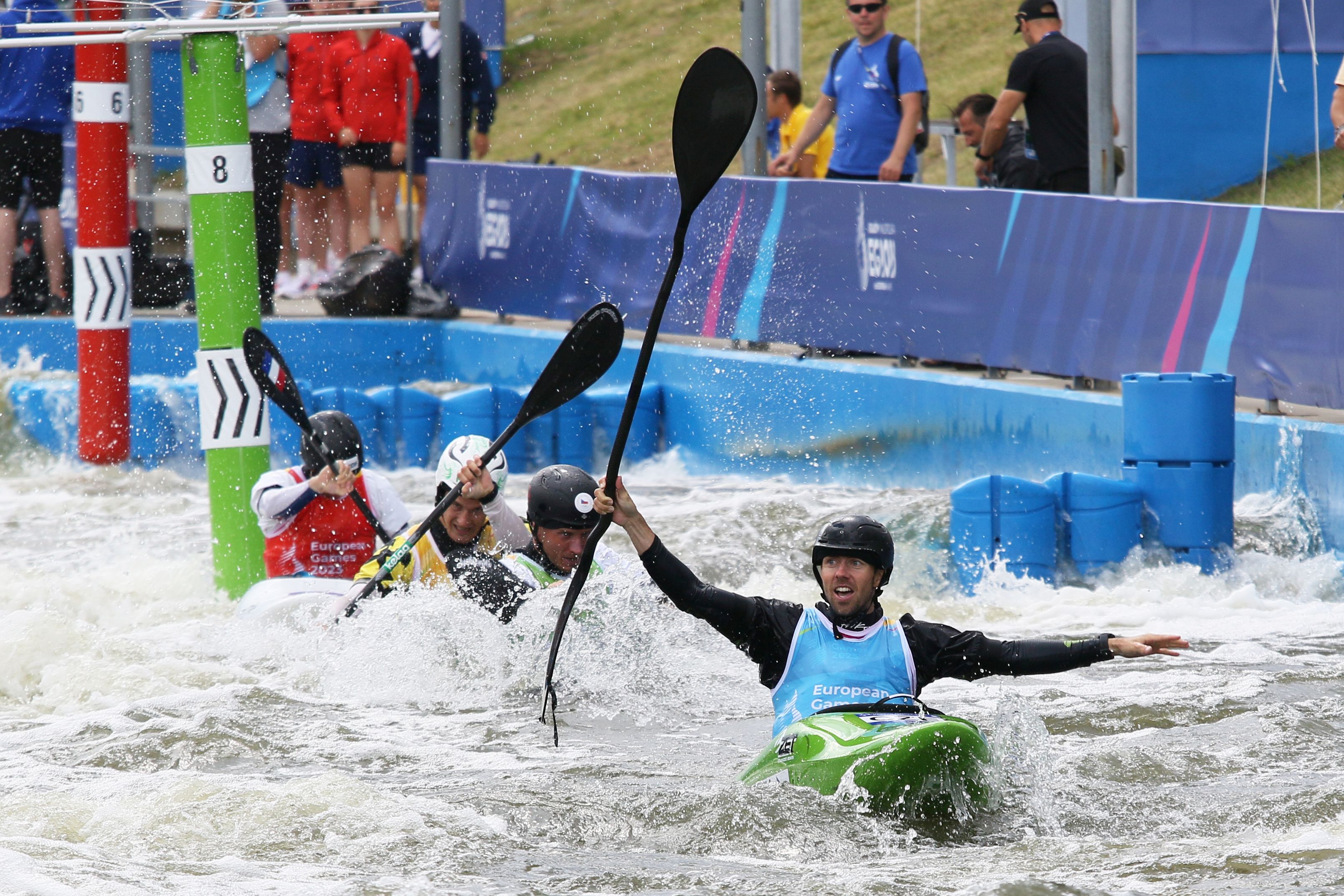This vivid, outdoor color photograph captures an intense moment from a kayak race, featuring four kayakers navigating a man-made river with blue concrete side walls and churning rapids. The lead kayaker, positioned prominently in a green kayak, is raising his paddle in a triumphant gesture, evidently having won the race. Three other kayakers, closely bunched together, trail behind him. All participants are equipped with black paddles and helmets for safety, with the trailing kayakers wearing black and white helmets respectively. The backdrop showcases a grassy hill dotted with spectators lined up behind what appears to be a plastic barricade. In this dynamic scene, the numbers "8" and "6" are visible on poles anchored in the water near the kayakers, adding a layer of competitive context to this thrilling race.